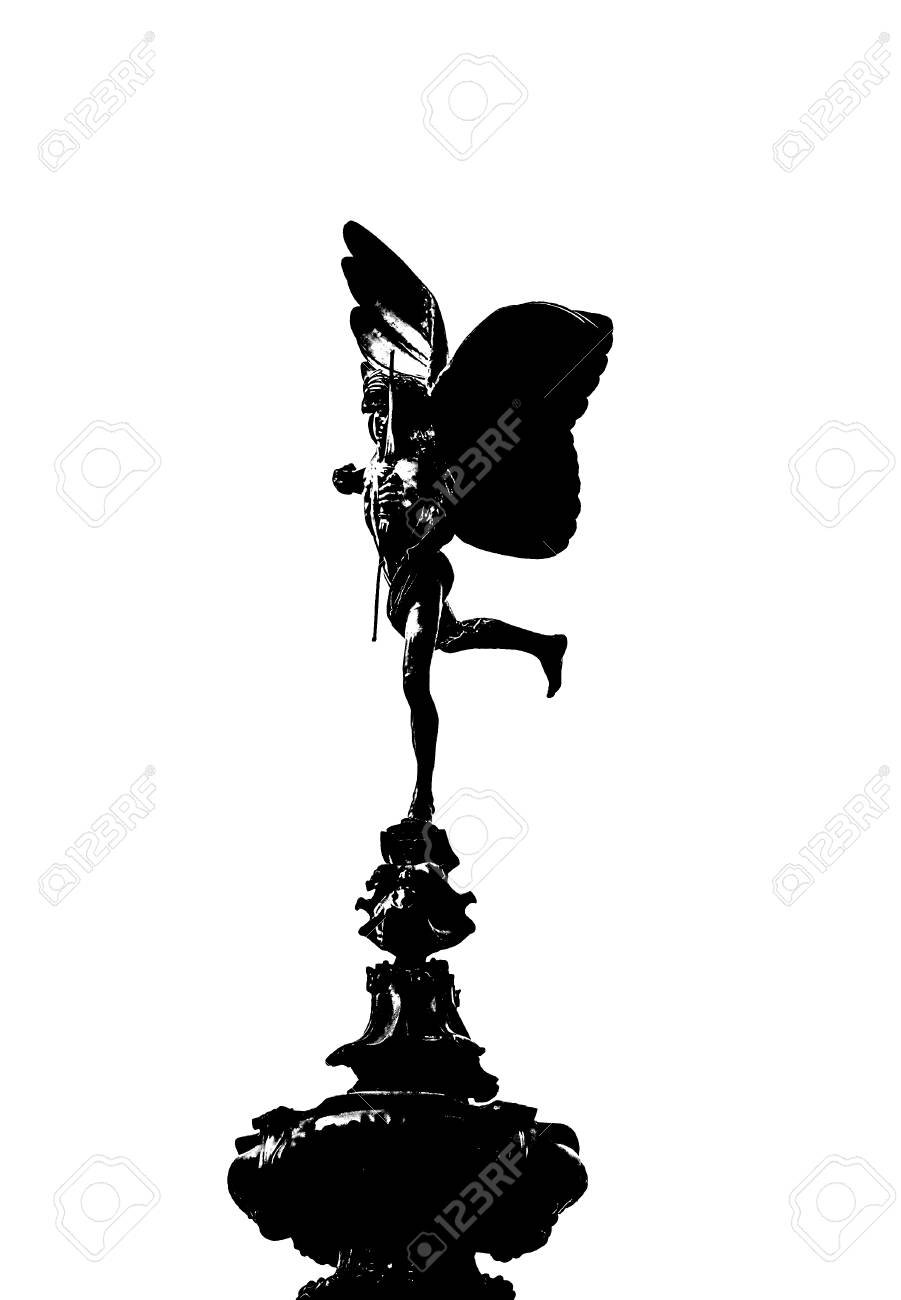The image features a black statue of an angelic figure with large, outstretched wings that rise higher than its head. It is depicted in a glossy finish, giving it a shiny appearance that reflects light. The angel, viewed from a side perspective, is poised gracefully on one leg, with its right leg kicked up behind it and standing tiptoe on a vase-like, floral base that resembles a fountain. The figure, which is thin and elongated, holds something in one of its hands that resembles a gavel or weapon. It is a black and white image, predominantly dark in tone, and watermarked with the text "123RF." The figure's wings evoke a delicate, almost butterfly-like quality, contributing to the artistic and ethereal essence of the sculpture.